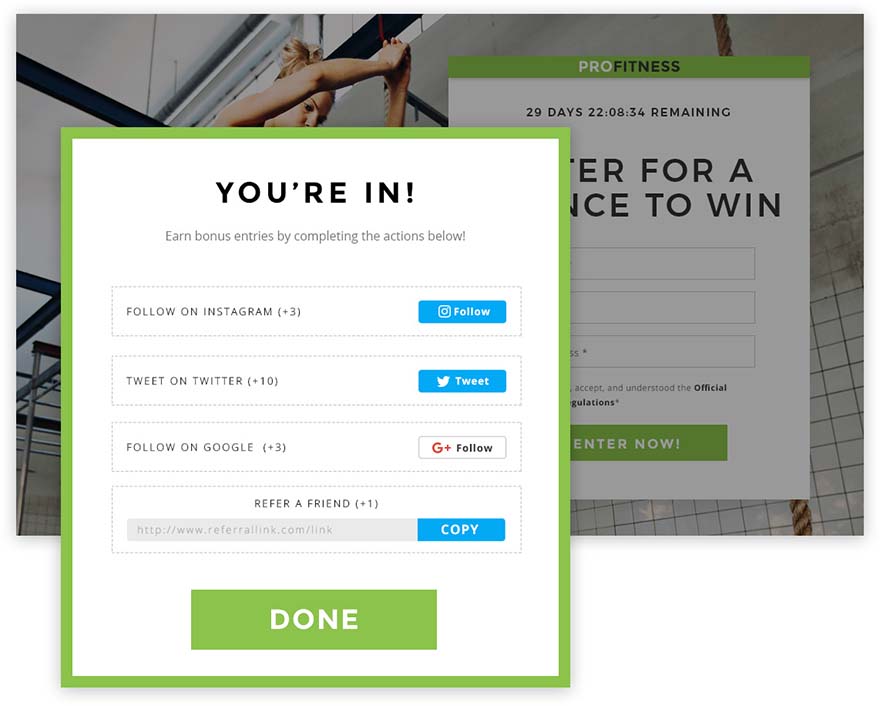In the image, a person with their hair styled in a bun is seen standing in front of a window, pressing their hands against the glass. The background appears to have a tiled pattern or a grated design, with cables and bars visible at the top. 

Intricately detailed green borders frame the main elements of the composition, including various call-to-action prompts and social media engagement indicators. Text prompts like "Share your aim" and "Aaron Post sent you a speck of a nice glow" are prominently displayed. There are multiple engagement metrics, such as "Follow on Instagram, +3," "Twitter +10, Tweet," "Follow on Google, +3, Instagram, follow," and "Refer a friend, +1."

A clean, green rectangle labeled "Enter Now" is positioned on the image, and several input fields are available for interaction. Additionally, there's a promotional callout for "Perl Fitness" indicating that users have 29 days remaining out of a specific period, with "22" days clearly highlighted for the chance to win something. An input field appears underneath this section for users to enter their details. The overall setting gives a sleek and interactive feel, underlined by modern visual elements and social media integration.